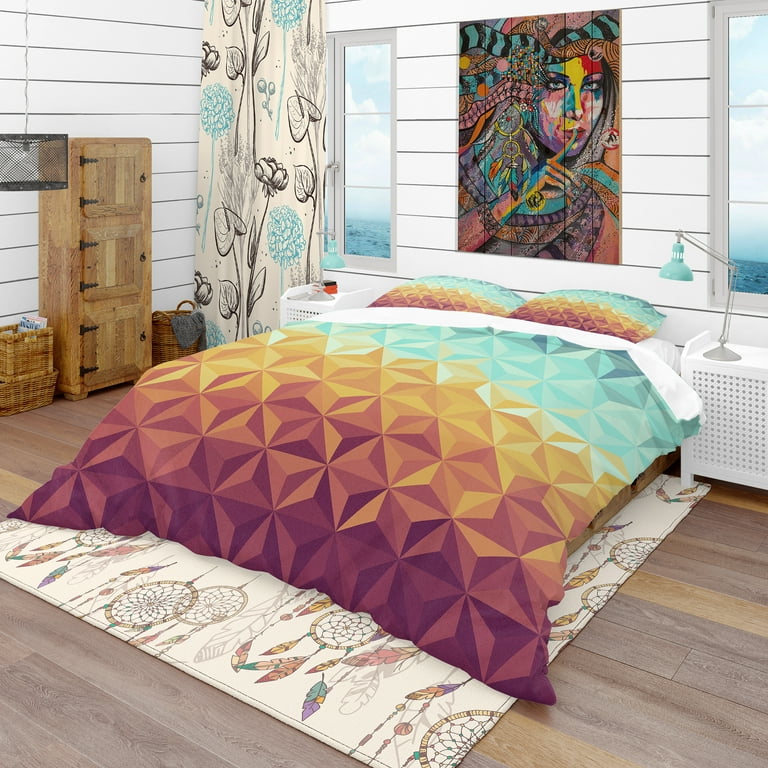This image depicts a meticulously designed bedroom, showcasing an interior designer's concept of an attractive and harmonious space. Dominating the scene is a full-size bed positioned against a backdrop of horizontal white shiplap planking. Notably, the bed lacks both a headboard and a footboard, allowing the geometric patterns on the bedding to stand out. The comforter and matching pillowcases feature an array of triangles and polygons in a striking palette that transitions from shades of green through orange to a deep, rich red.

Above the bed, a captivating work of art displays a Middle Eastern woman adorned in jewels and a resplendent gown, her face painted with vibrant colors such as red, yellow, green, and blue. She holds her hand over her mouth, conveying a sense of quiet or whispering. 

Flanking the bed, two white nightstands are topped with mint-colored gooseneck lamps, providing a pop of color against the otherwise neutral hues. The bed sits atop a beige area rug decorated with dreamcatcher motifs, resting on medium-toned wooden floorboards that add warmth to the room.

To the left, a beautiful wooden three-door chest contributes additional storage, while wicker baskets and enclosures for possible radiant heaters are neatly arranged to the right. The room also features beige vertical drapes adorned with a black and mint floral pattern, echoing the artistic designs found in the throw rug beneath the bed. The windows framing the bed offer a glimpse of a cold exterior, contrasting with the cozy, inviting atmosphere of the room.